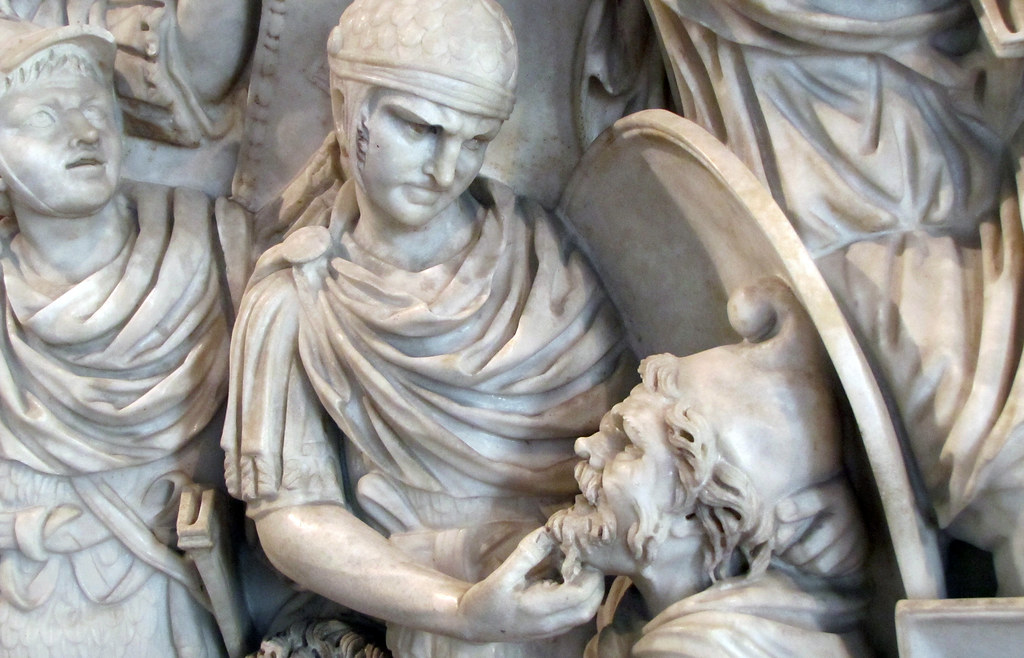This photograph showcases a detailed close-up of a marble sculpture from a sarcophagus dated around 250 AD, depicting a dramatic scene likely related to war. The central figure, a Roman military leader, is adorned in traditional Roman garb, wearing a helmet and a flowing robe. He holds a shield and is captured in a striking pose as he grips the chin of an older, bearded man positioned lower than him, whose expression appears a blend of fear and anger. This older man, also wearing a cap, has the central figure's other hand placed firmly on the back of his head. To the left, a third figure, also in traditional attire and seemingly engaged in the scene, looks upwards with slightly parted lips. The sculpture is intricately carved from white marble, vivid in its depiction of the figures' clothing and expressions. While the central three figures are prominently visible, additional soldiers appear in the background, their forms partially obscured and rendered without detailed facial features, adding to the crowded and chaotic ambiance of the portrayed battle.